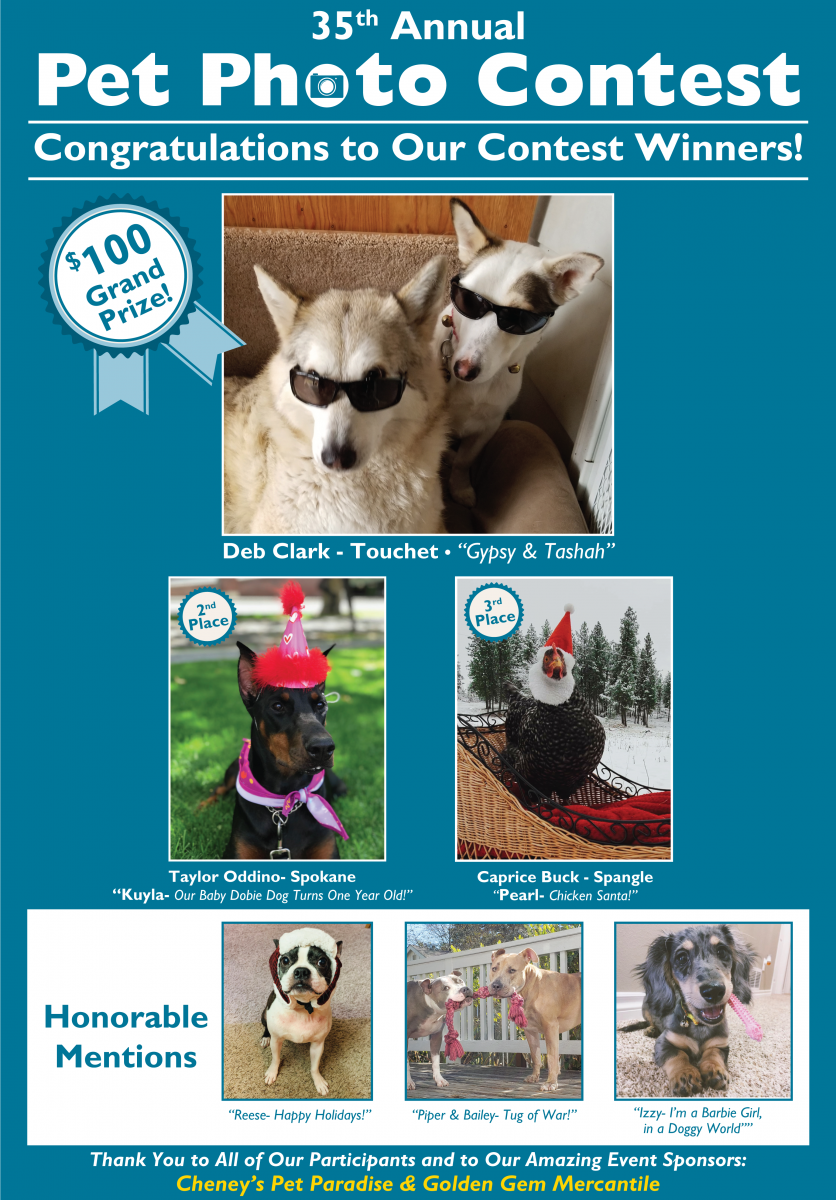The flyer features the 35th Annual Pet Photo Contest on a lovely sky-blue background. At the top, it proudly announces "Congratulations to our contest winners!" A ribbon in the upper left corner states "$100 Grand Prize," which was awarded to Deb Clark of Touche for her photo of two dogs, Gypsy and Tasha, wearing sunglasses while lounging on a couch. 

Below the grand prize image are the second and third place photos. Second place, awarded to Taylor Adino of Spokane, showcases Koila, a Doberman wearing a birthday party hat and a purple bandana, lying on the grass. Third place, awarded to Caprice Buck of Spangle, features Pearl the Chicken dressed in a Santa hat, enjoying a winter scene in a sleigh.

At the bottom of the poster are the honorable mentions: Reese, a dog sitting and looking up; Piper and Bailey, two dogs engaging in a playful tug-of-war with a toy; and Izzy, a dog happily smiling. 

The footer of the poster expresses gratitude: "Thank you to all of our participants and to our amazing event sponsors," listing Cheney's Pet Paradise and Golden Gym Mercantile.